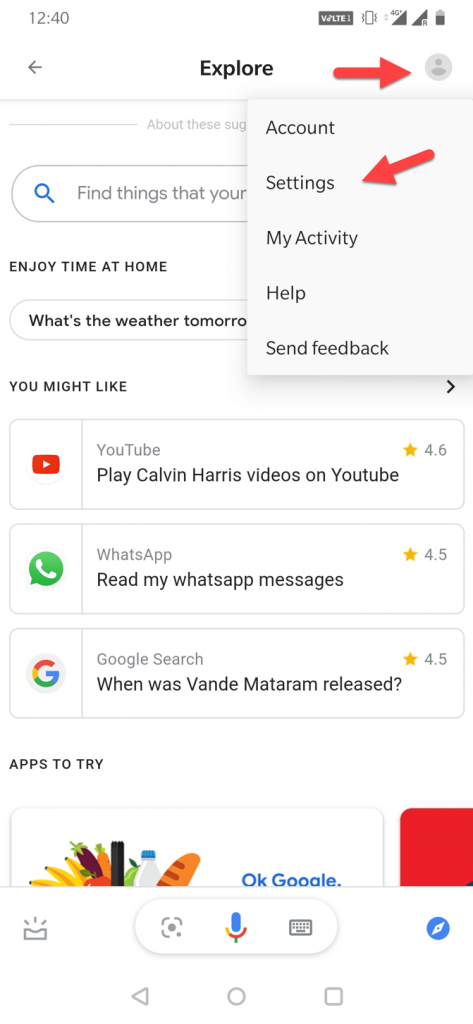This image is a screenshot taken from a cell phone screen. The main background of the image is white, and at the top, the word "Explore" is prominently displayed in black print. In the upper right-hand area of the image, there is a pop-up box, digitally annotated for explanatory purposes.

A red arrow points to a circular icon featuring a silhouette of a person, indicating user profile-related options. Below this icon, within the pop-up box, there are several menu options listed: "Account," "Settings," "My Activity," "Help," and "Send Feedback." Another red arrow directs attention to the word "Settings" within this menu, contrasting the first arrow by pointing leftward and slightly downward.

Further down the page, the text "Find Things that You're" is visible in black print, followed by additional text, "Enjoy Time at Home," and a clickable item stating, "What's the weather tomorrow?" 

The section labeled "You Might Like" showcases three app suggestions: YouTube, WhatsApp, and a Google search icon. At the bottom of the image, the text "Apps to Try" is partially visible but appears to be cut off. The red arrows and menu labels suggest that the image serves an instructional or tutorial purpose.